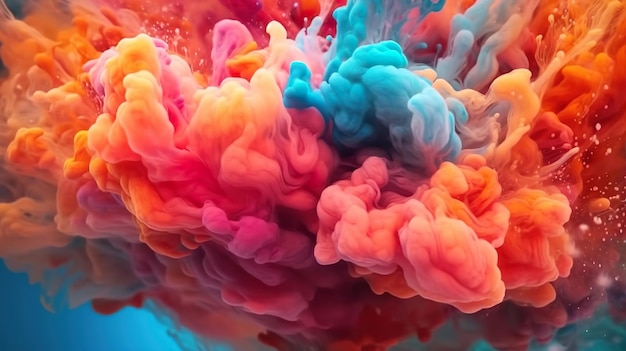The image is a stunning, close-up photograph of colorful, cloud-like formations that resemble puffs of smoke or dye injected into water. The vibrant display consists of separate, soft, and floaty colors that look like they are suspended in a clear blue liquid, enhancing the impression of underwater phenomena. Dominant colors include vivid fuchsia, brilliant blue, bright orange, soft peach, creamy yellow, and hints of purples and pinks. Each color maintains its integrity without blending into others, creating distinct, wave-like structures that give the impression of cotton candy or delicate loofah textures. The edges of the formations appear to splatter slightly, adding to the dynamic and ethereal quality of the scene. This mesmerizing interplay of colors and textures makes the image extraordinarily beautiful and visually captivating.